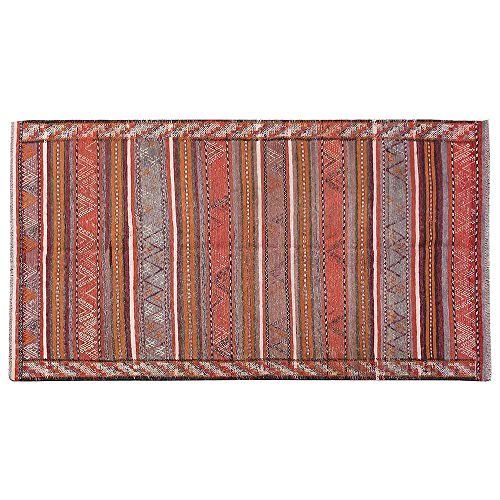This rectangular rug features an intricate and vibrant design composed of a variety of patterns and colors. Dominant hues include red, light gray, gray-blue, brown, white, and orange. The center section of the rug boasts vertical white stripes and thin red stripes interspersed with small circles on an orange background. Brown stripes add to the complex design within this central region.

The border of the rug is equally elaborate, with diagonal quilted patterns integrating red, gray, orange, and brown. The longer sides of the rug feature alternating stripes of red and bluish-white, while the shorter sides are adorned with alternating orange and white triangles.

In between the borders, the rug displays diverse motifs such as checkered lines in black and white or white and gray, and repeating dotted patterns with white dots on an orange background. Additionally, triangle patterns and gray shapes resembling mountains further enrich the central zone, creating a tapestry of continuous, repeating designs.